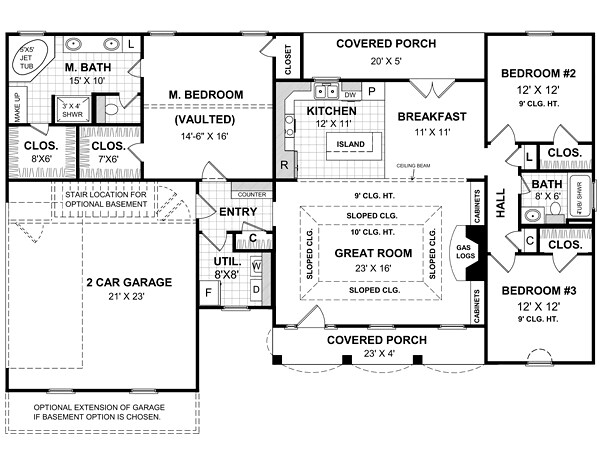This architectural floor plan features a detailed layout on a white background with black lines and annotated text indicating the names and dimensions of various rooms. In the upper left corner, the master bedroom suite includes a master bathroom measuring 15 feet by 10 feet and two closets, one measuring 8 feet by 6 feet and the other 7 feet by 6 feet. Directly below the master suite is a spacious two-car garage, which spans 21 feet by 23 feet. Adjacent to the master bedroom on the right is a covered porch. Below the covered porch lies the kitchen and breakfast room area. In the upper right quadrant, the second bedroom, complete with an attached closet, measures 12 feet by 12 feet. A small hallway connects to the second bathroom and leads to the third bedroom situated at the bottom right corner of the house. Central to all of these spaces is a great room, which serves as the focal point of the layout. Additionally, there is a second covered porch located at the bottom of the plan.